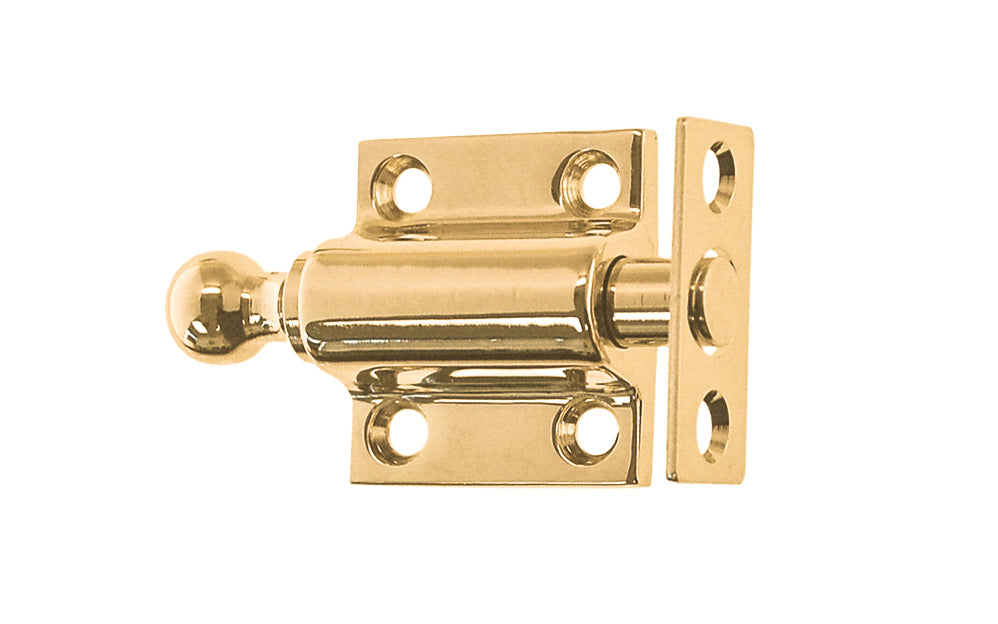This is a very detailed close-up image of a shiny, gold-colored sliding door lock, prominently set against a completely white background with no other objects. The lock is square in overall shape but features a cylindrical curve on a hill. The cylinder, located inside the lock, has a handle on the left side that resembles a small doorknob or round ball, reflecting light and possibly the room's surroundings. There are six bolt holes in total: four on the rectangular backplate—two at the top and two at the bottom—and two additional holes on the cylindrical part. The entire structure is very shiny, allowing reflections to be seen across its surface. Additionally, a noteworthy detail includes a gold pin mechanism that slides in and out for locking, with a distinct gold ball top. The image offers a detailed view from a corner perspective, showing both the front and side of the lock, and capturing intricate details such as rivets, grooves for screws, and various small components of the locking mechanism.